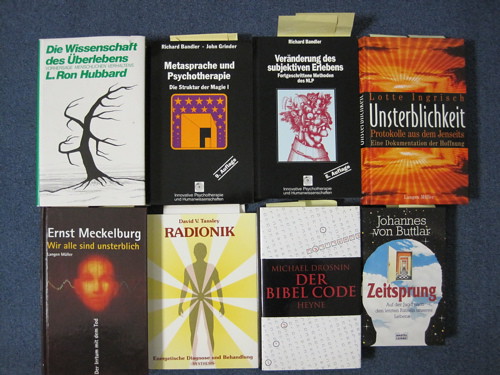A top-down photograph shows eight hardbound books arranged on a blue surface, most of which are in German. The first book, "Die Wissenschaft des Überlebens" by L. Ron Hubbard, features a barren black tree on a white cover with green text. Another book, "Metasprock and Psychotherapy," has a black cover with an orange square, orange stars, and additional purple decor. A black book with a white banner displays red flowers. An orange and black book presents an illustration of a sunset. There is also a book featuring a man's face on a muted red and black cover, captioned "Unsterblickeit" by Ernst Mecklen. Additionally, a yellow book with radial yellow and white stripes and a silhouette of a man is titled "Radionik." Another book is white with a black rectangle and red text, titled "Der Bibelcode." The final book has a black cover with an outline of a head leading to a door on a checkered floor, and clouds inside the head, titled "Sieg Sprung." Some books have yellow post-its or place markers sticking out from the tops.